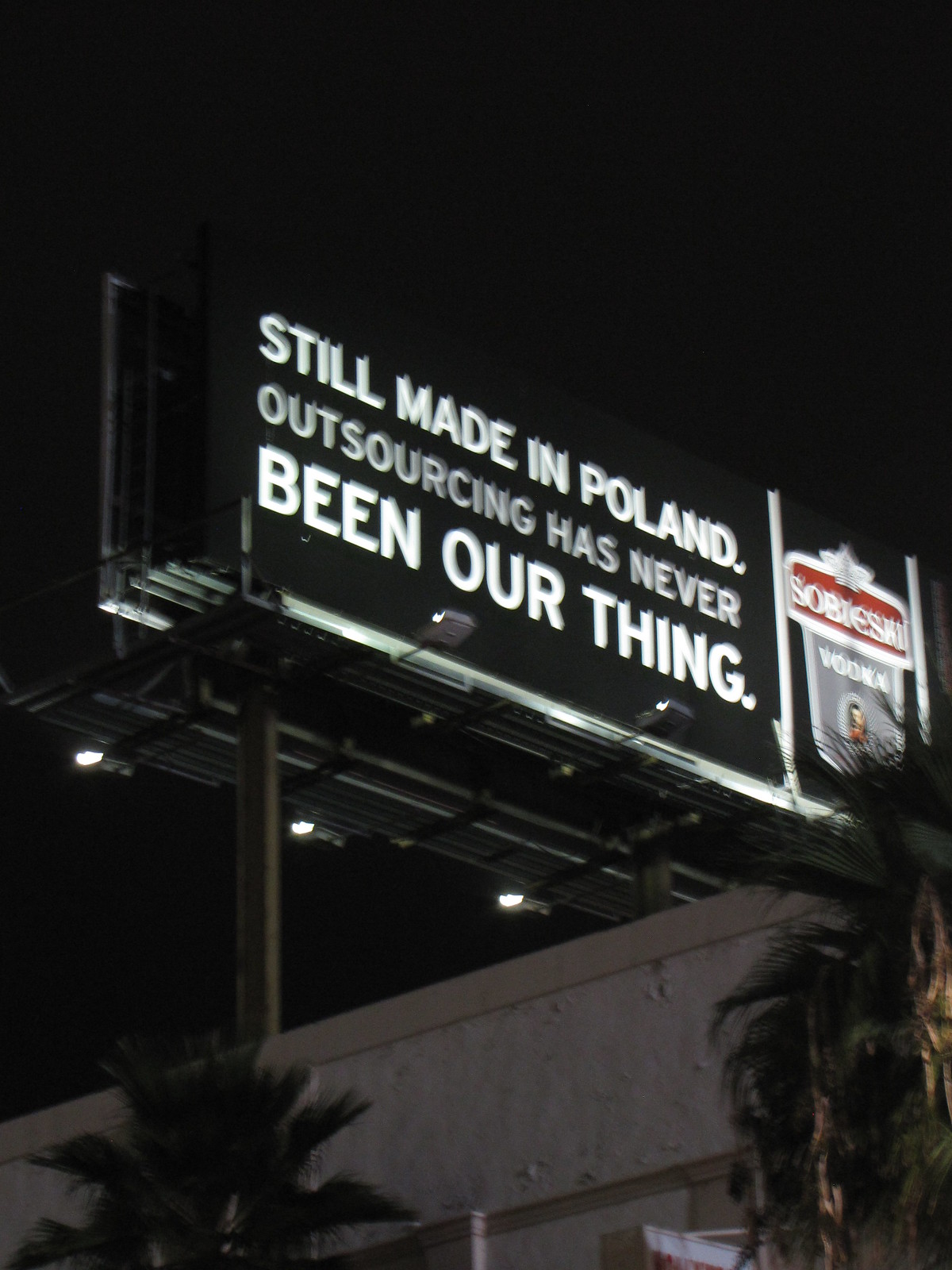The image depicts a vertically-oriented rectangular billboard with a sleek black background. Occupying approximately three-quarters of the left side of the billboard is a bold white statement: "Bill made in Poland. Outsourcing has never been our thing." On the right side of the billboard, taking up the remaining space, are the words "Sobieski Vodka" accompanied by an oblong-shaped emblem. The billboard is illuminated by lights positioned at the bottom, casting a glow upwards to ensure it is visible even in low-light conditions. The billboard itself is mounted on a flat support system and anchored by two sturdy poles. Below the billboard, a building and a few palm trees can be seen in the background, adding to the urban landscape of the scene.